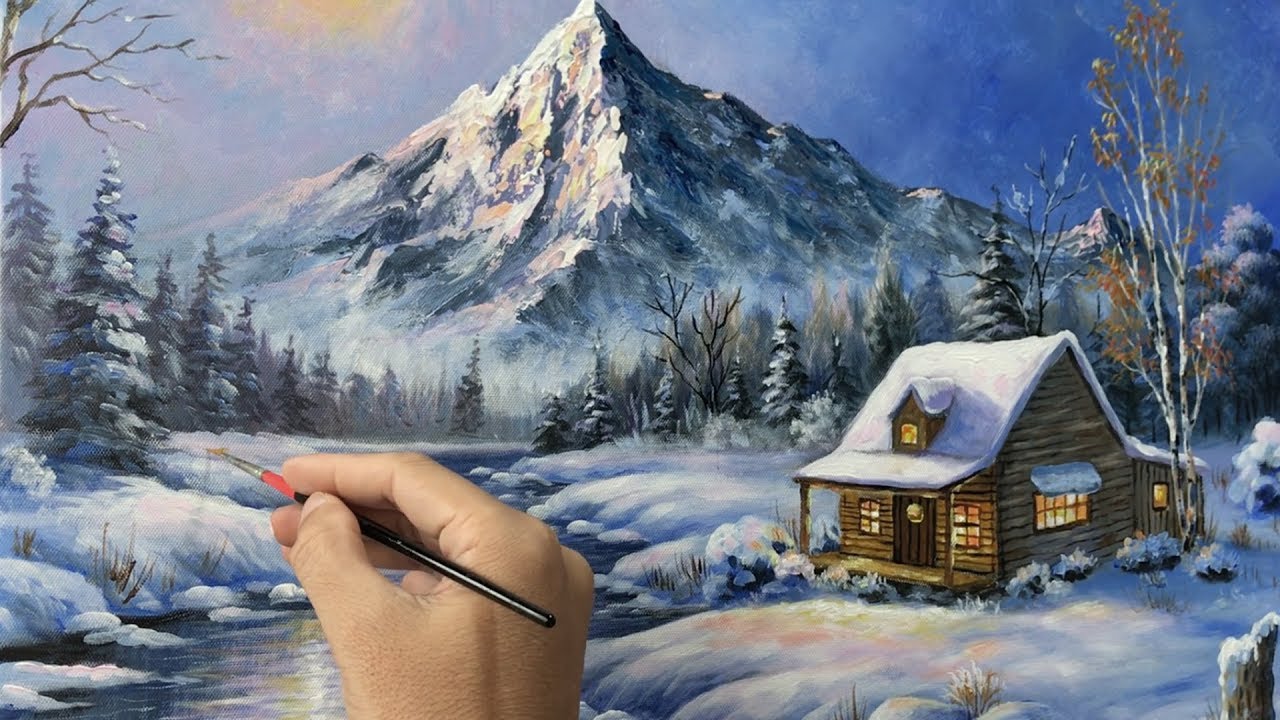This image captures a right-handed person with light skin, holding a paintbrush with a black handle, silver ferrule, and a pink upper section, meticulously painting a winter scene. The painting, reminiscent of Thomas Kinkade's style, features a cozy snow-covered cabin to the right, illuminated with lights that cast warm pink and yellow hues onto the surrounding snow. In the center background, a majestic mountain rises, framed by a vibrant blue sky with a low-set sun. The foreground shows a series of declining Christmas trees on the left, some branches, and a meandering creek close to the cabin reflecting the sunlight. The entire scene is blanketed in snow, capturing the serene beauty of a winter landscape.